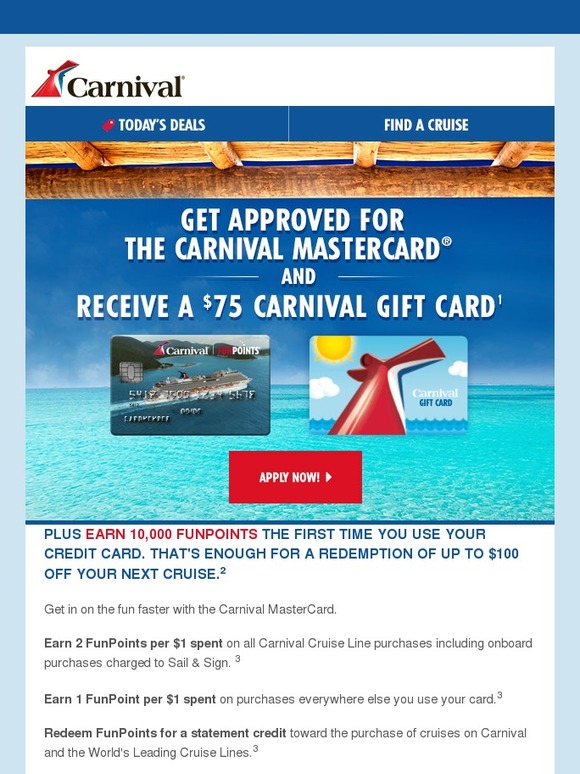**Caption:** 

A cropped screenshot from a carnival website showcasing the "Today's Top Deals" page. The header features a dark blue bar, with the main background in light blue. A large white square is prominently centered on the page. At the top left of this square, the 'Carnival' logo is displayed. Below the logo, two blue bars serve as navigation tabs – “Today's Deals” on the left and “Find a Cruise” on the right.

The focal content displays a serene image of crystal blue ocean waters. Above this image, bold text reads: "Get Approved for the Carnival Mastercard and Receive a $75 Carnival Gift Card." To the left of this text is a thumbnail of the Carnival Credit Card, with a thumbnail of the Carnival Gift Card to the right. At the bottom center of the content, a red rectangle marked "Apply Now" with an arrow pointing left serves as a call to action. Below this, an informational footer reads: "Details. You earn 10,000 Fun Points the first time you use your credit card. That's enough for a redemption of up to $100 off your next cruise."